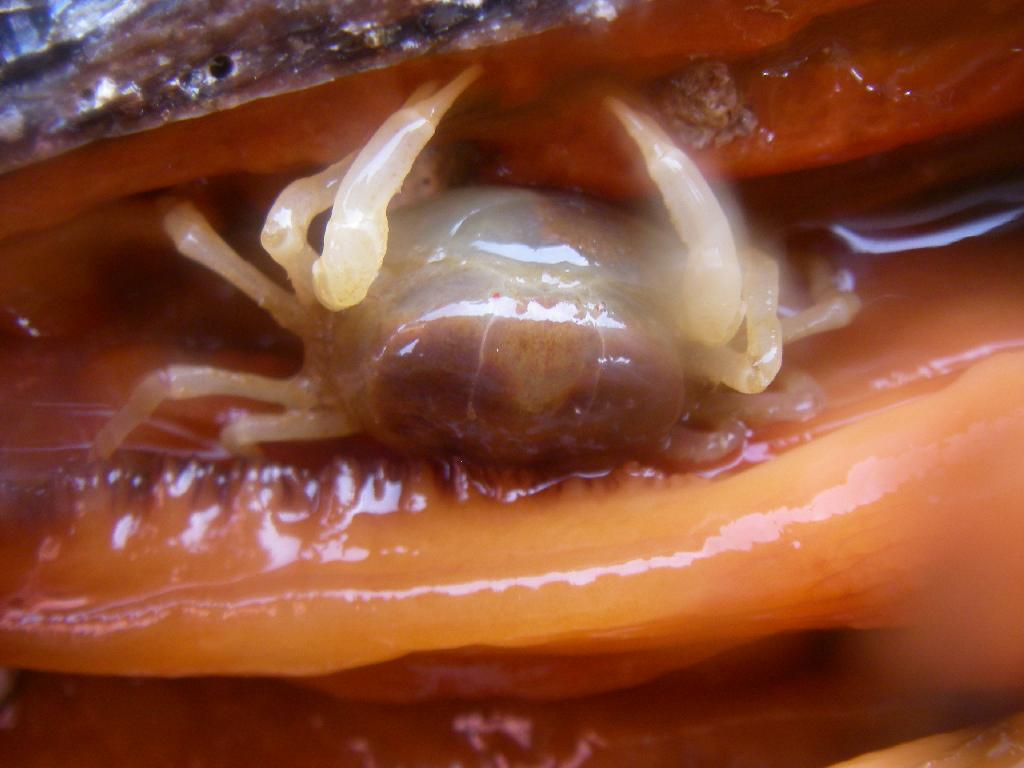This photograph is a detailed, close-up shot of a pea crab nestled within what appears to be a clam shell. The transparent, almost luminescent crab features see-through legs and pincers, while its main body is an opaque white, slightly darker on the underside. The crab is surrounded by a mucous-like, wet environment, likely the soft, pink meat inside the clam shell. The surrounding area within the shell displays hues of orange and peach, adding to the distinctive setting. Often considered an unwelcome pest, this tiny, translucent crab, with its delicate and clear limbs, sits against the backdrop of the slimy, orange-toned interior of the shell.